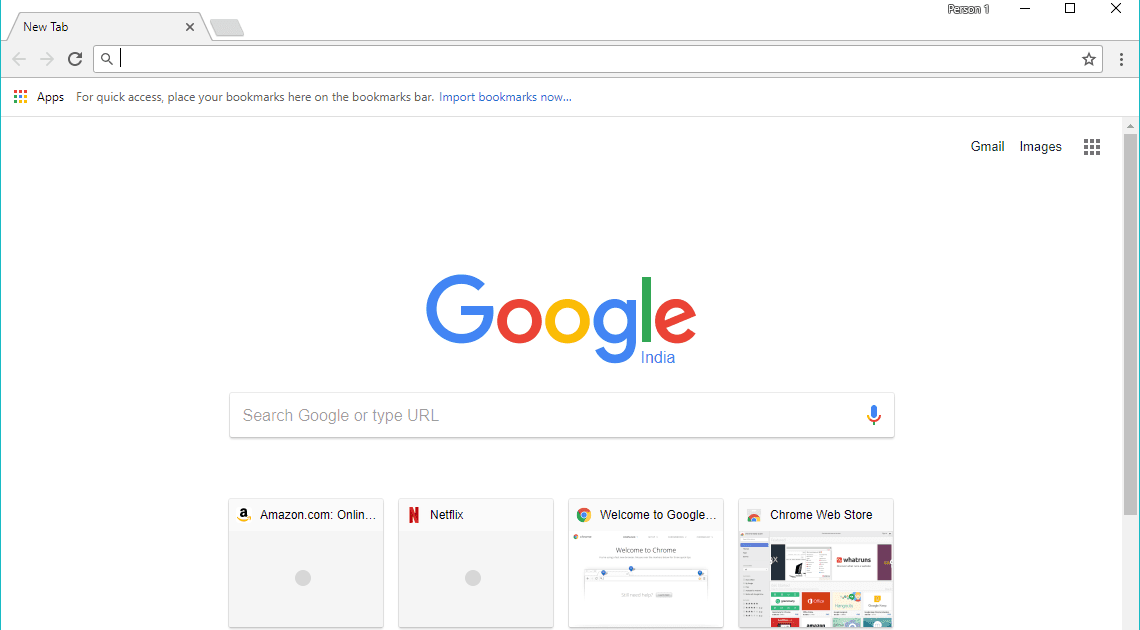This is a detailed screenshot of the Google India homepage. The top section features an empty search bar with a prompt encouraging users to add bookmarks: "Place your bookmarks here on the bookmarks bar. Import bookmarks now." Adjacent to this section, on the top-right side, there are icons and text for "Gmail" and "Images," along with a grid icon composed of three rows of three dark squares, signifying Google apps.

The main body of the webpage is set against a white background and prominently displays the Google India logo centered on the page. The Google text is illustrated with its iconic colors: the first "G" is blue, the first "O" is red, the second "O" is yellow, the second "G" is blue, the "L" is green, and the "E" is red. Below the "L" and "E," the word "India" is written in blue letters.

Beneath the Google logo, there is a search bar with the placeholder text "Search Google or type URL" and a microphone icon on the far right, indicating voice search capability. Under the search bar, there are four windows, each with different labels: "Amazon.com," "Netflix," "Welcome to Google," and "Chrome Web Store."

The webpage is devoid of any human, animal, or plant imagery, maintaining a clean and minimalistic design.